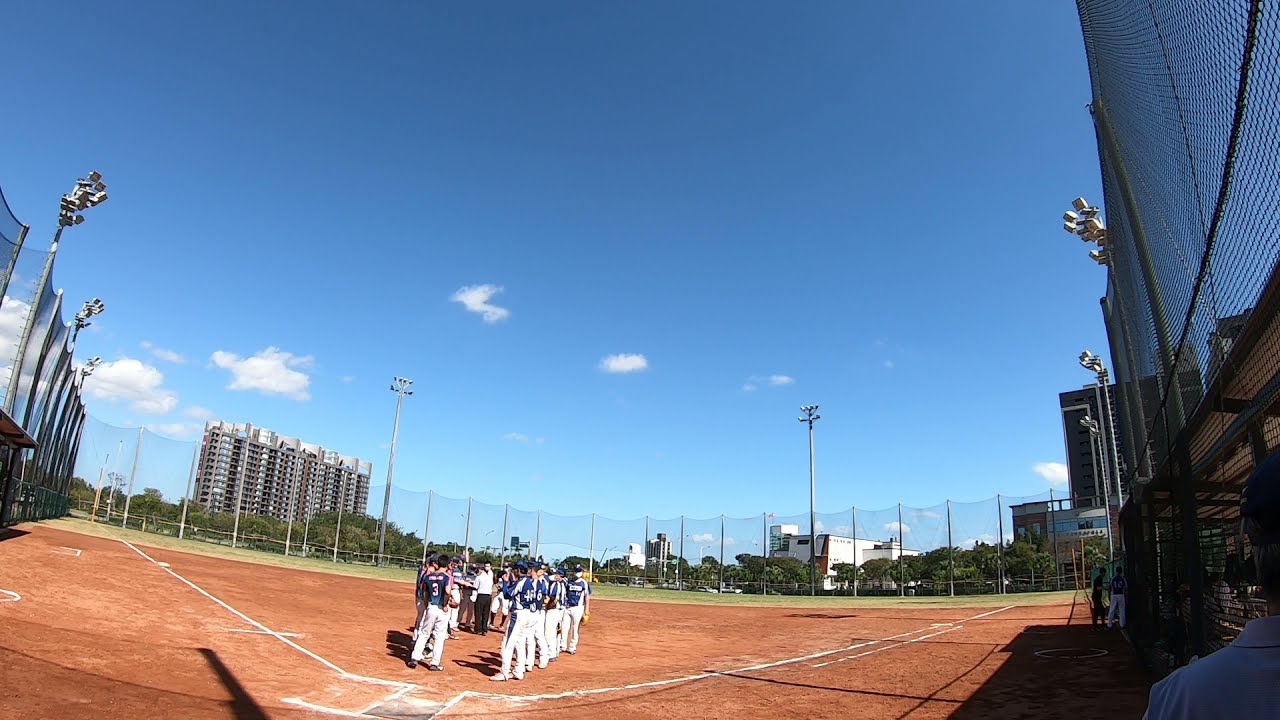In this vibrant photo of a baseball field, a group of boys is captured standing in lines near home plate, dressed in matching blue jerseys and white pants. The scene is viewed from behind the catcher, highlighting the netting fence that encapsulates the field. In the middle, a man stands among the boys, possibly orchestrating a post-game handshake or assembly. Beyond the field, tall poles with lights frame the area, and a tall building structure looms in the distance alongside some trees. The sky above is a brilliant blue with only a few scattered clouds, underscoring the bright, sunny day's clarity and adding to the cheerful atmosphere.